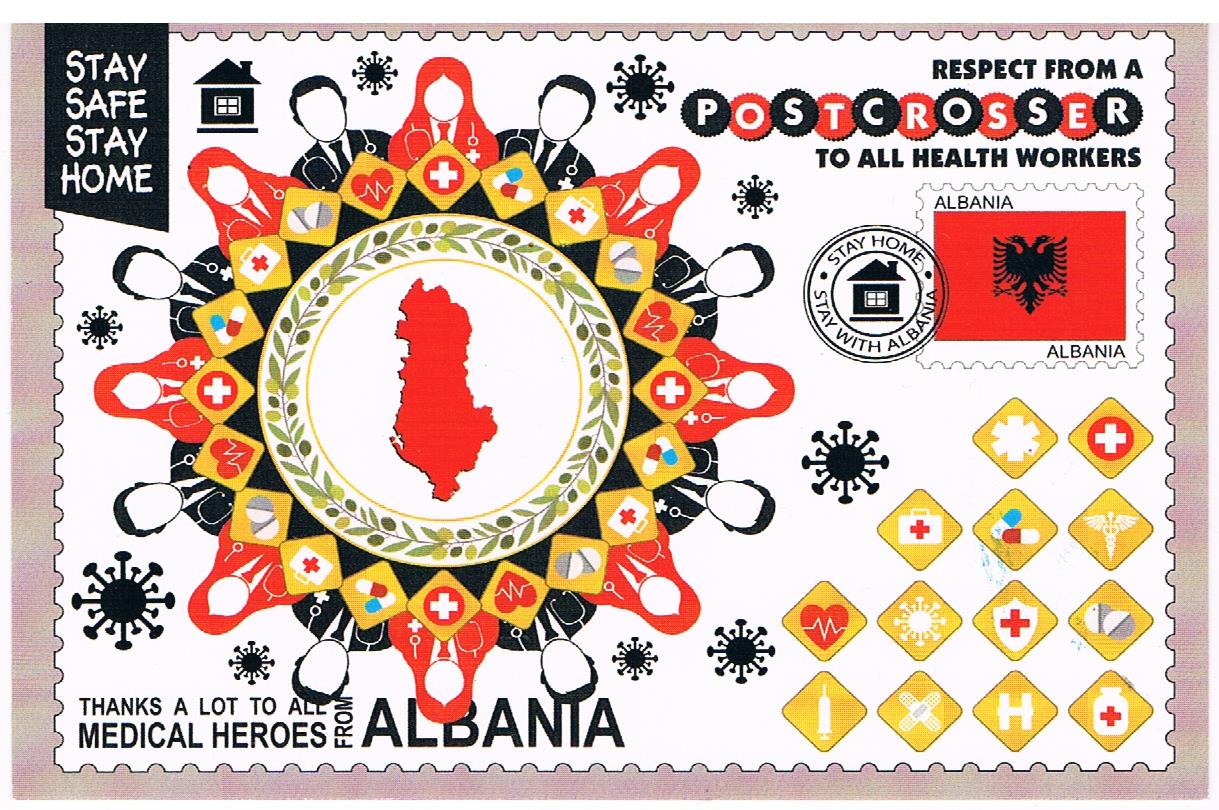The postcard, titled "Respect from a Post-Crosser to All Health Workers," is a detailed and colorful homage to medical workers, presumably released by Albania during a pandemic. The rectangular postcard features a predominantly white background with vibrant red, black, yellow, pink, and green elements.

Encircling the central design is a plaid border in pink and green hues. The central focus is Albania's map, symbolizing the origin of this tribute. Surrounding this nucleus is a wreath-like floral pattern, further encased in yellow diamond-shaped boxes containing iconic medical symbols such as a cardiogram, aspirin tablets, a first-aid kit, a syringe, band-aids, and the Red Cross badge.

Additionally, there are alternating faceless headshots of long-haired figures in red and short-haired figures in black, each adorned with stethoscopes, symbolizing both male and female healthcare workers. This alternating pattern provides a visual representation of the workforce.

In the top left corner of the postcard, there is white text on a small rectangle that reads, "Stay Safe, Stay Home." The top right corner bears the message, "Respect from a post-crosser to all health workers" in black text. The bottom left corner thanks medical heroes with the note, "Thanks a lot to all medical heroes from Albania." An image of the Albanian flag, with "Albania" inscribed above and below it, is also prominent beneath the top-right message.

Overall, this postcard serves as a multi-faceted tribute to healthcare professionals worldwide, merging visual elements and text to express gratitude and solidarity amidst a global health crisis.